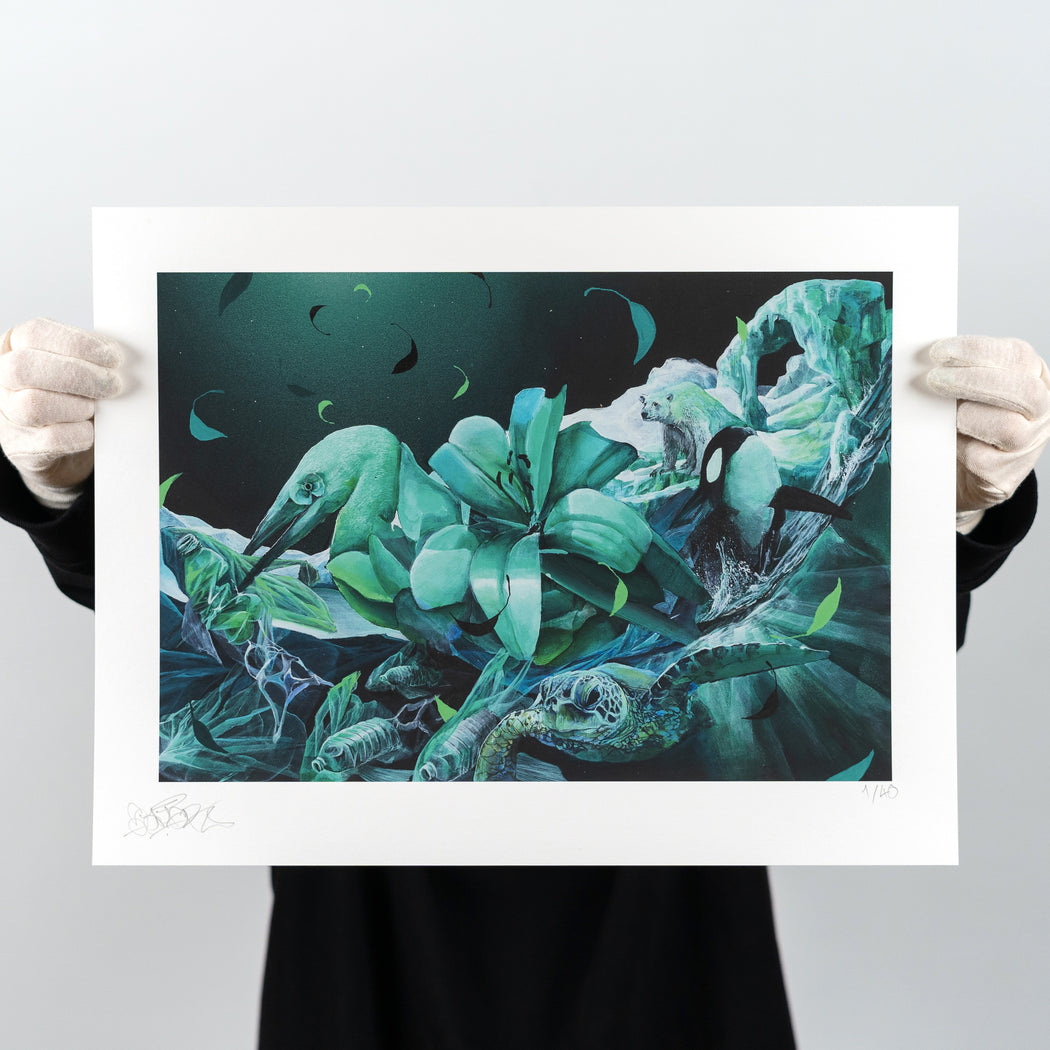A person dressed in a long black sleeve shirt and white cloth gloves is holding an elaborate art print. The print, which they handle carefully by its white matting, completely obscures their face, being held at chest to face level. The print is rich in details and mostly showcases various shades of green, black, and blue-green in a near-monochromatic palette. It features an intricate combination of flora and fauna, with deep green floral designs, different types of plant life like iris plants, and foliage with thick green petals. The image includes a swimming sea turtle with its legs extended, various birds resembling herons or large sea birds with small fish in their beaks, as well as polar bears, orca whales, and even coral. Trash floating in the water deftly hints at environmental themes. The upper left corner of the print offers an underwater view with leaves flowing through water. This evocative and detailed print combines both terrestial and marine elements, suggesting a broader ecological message.